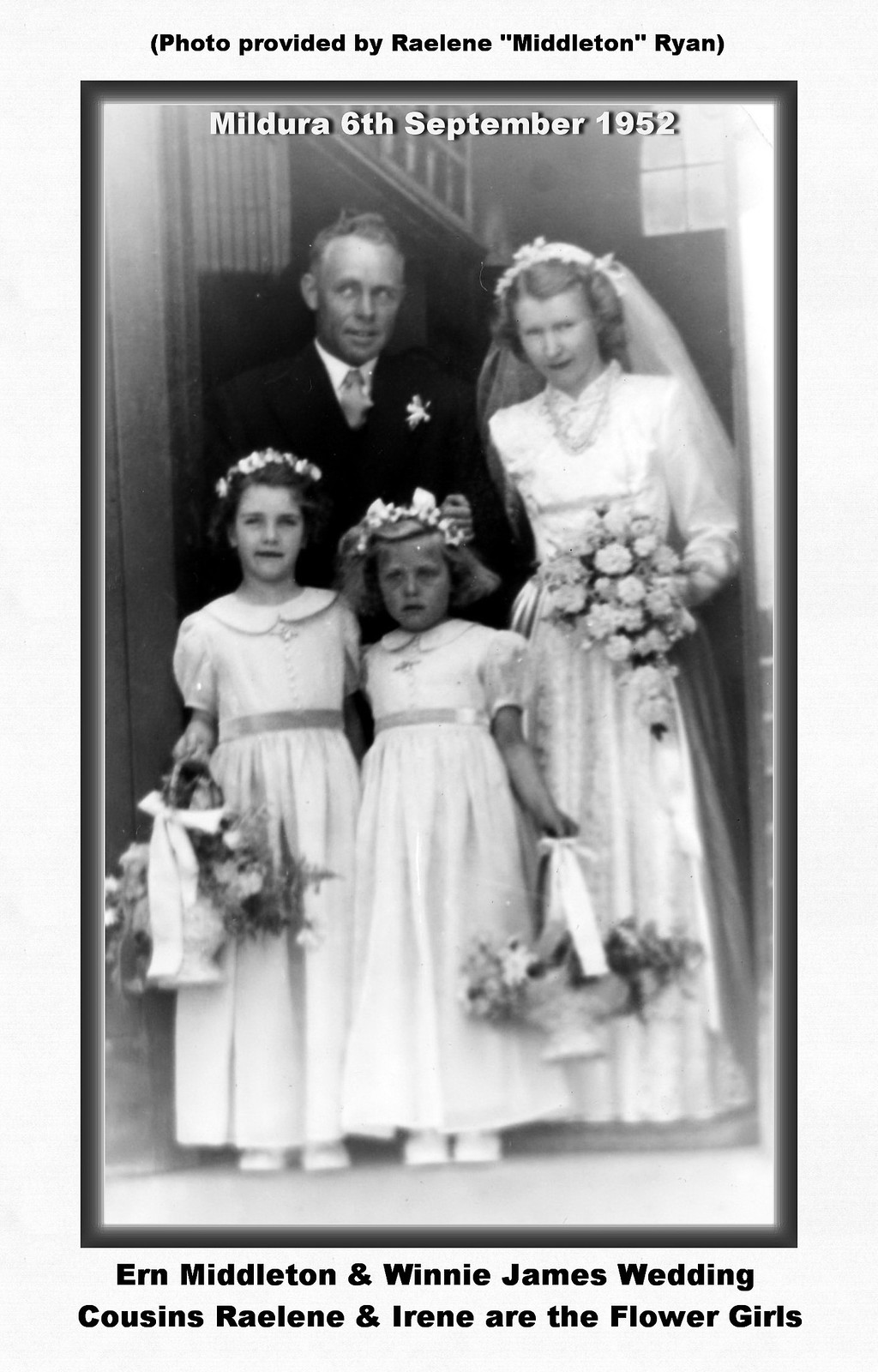This detailed black-and-white wedding photograph, dated 6th September 1952, taken in Mildura, captures a momentous family event. The image, provided by Raylene Middleton Ryan, shows four people standing at what appears to be the entrance of a church. 

The groom, Erne Middleton, is dressed in a dark, buttoned-up suit with a tightly fastened tie and a boutonniere on his left breast. He has short, light brown hair and is gazing to his right. Standing next to him is the bride, Winnie James, slightly shorter than the groom, with curly light brown hair and a delicate veil cascading over her shoulders. She is adorned in a long, white wedding gown with intricate floral designs and holds a bouquet of white flowers in her bent left arm.

In front of the couple are two young flower girls, identified as cousins Raylene and Irene. They are dressed in white dresses with ribbons around their chests and floral headbands adorning their heads. Each girl carries a small basket of flowers in one hand; one girl has brown hair, and the other appears to be blonde.

Behind the group, a staircase and a window are partially visible, establishing the church setting further. The top of the photograph bears the inscription "Mildura, 6th September 1952" in a white font, while the bottom reads "Erne Middleton and Winnie James Wedding" with a note identifying "cousins Raylene and Irene as the flower girls."